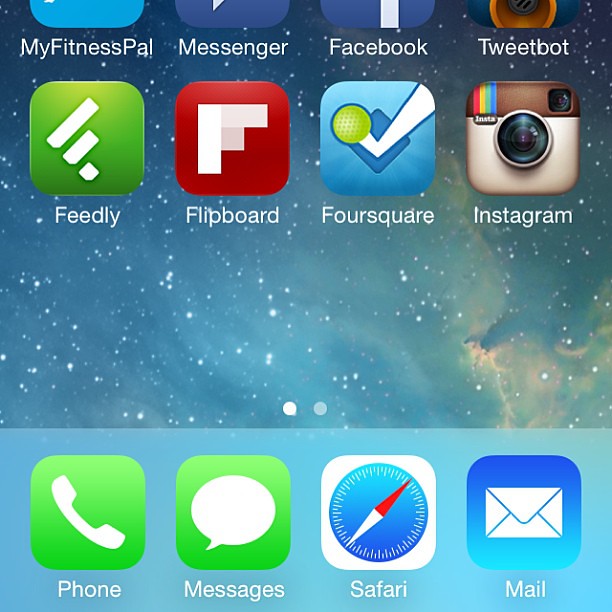The image shows a smartphone home screen with a variety of app icons arranged neatly. The top row of icons is slightly cut off, but you can discern the following apps from left to right: MyFitnessPal, Messenger, Facebook, and TweetBop. The second row features four apps, showcased with their distinct icon colors: Feedly (green and white), Flipboard (red and white), Foursquare (a mix of blue, green, and white), and Instagram, recognizable by its camera icon.

The background above these icons depicts an outer space scene with a deep blue hue speckled with white star-like dots. Below the app icons, you find the dock area with four more icons: Phone (green and white), Messages (green and white speech bubble), Safari (the iconic compass), and Mail (an envelope icon). This dock section has a lighter blue background, visually separating it from the celestial motif above.